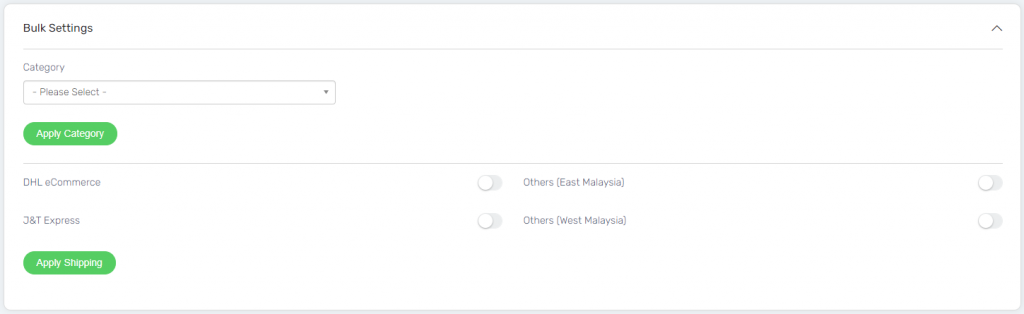Sure! Here is a cleaned up, descriptive caption for the image:

---

This image displays the 'Bulk Settings' section of a web page. The section features an expanded drop-down menu titled 'Category', below which there is another drop-down labeled 'Please Select'. Once an option is selected, users can apply a category using the respective apply button.

Following the category selection, the image shows options for shipping settings. The first option listed is 'DHL eCommerce', accompanied by a button labeled 'Others' with 'East Malaysia' indicated to its right. Another button, currently toggled off, is positioned beside it.

The second shipping option displayed is 'J&T Express', also with an 'Others' button followed by 'West Malaysia'. Similarly, there is a toggle button next to it that is off.

At the bottom, there is a button labeled 'Apply Shipping', allowing users to finalize their shipping choices for either East Malaysia or West Malaysia.

Overall, the 'Bulk Settings' section provides a clear interface for selecting categories and applying shipping options.

---